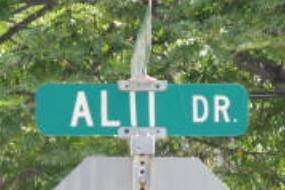The image depicts a somewhat low-resolution, slightly blurry thumbnail photograph taken outdoors. Central to the image is a green, elongated street sign prominently displaying the white text "Ali Drive." Above it, positioned perpendicularly, is another sign with text that remains unreadable. Both signs are mounted on a metal pole featuring adjustment knobs or recesses on the side. Below the main sign, the back of a large hexagonal sign, likely a stop sign, is visible along with light gray metallic fixtures and screws securing the signs in place. In the background, a canopy of trees with light and dark green leaves allows sunlight to filter through, creating a sun-dappled effect. The trees’ dark brown branches and some dark brown bark frame the scene, adding depth and contributing to the outdoor setting of the photograph.